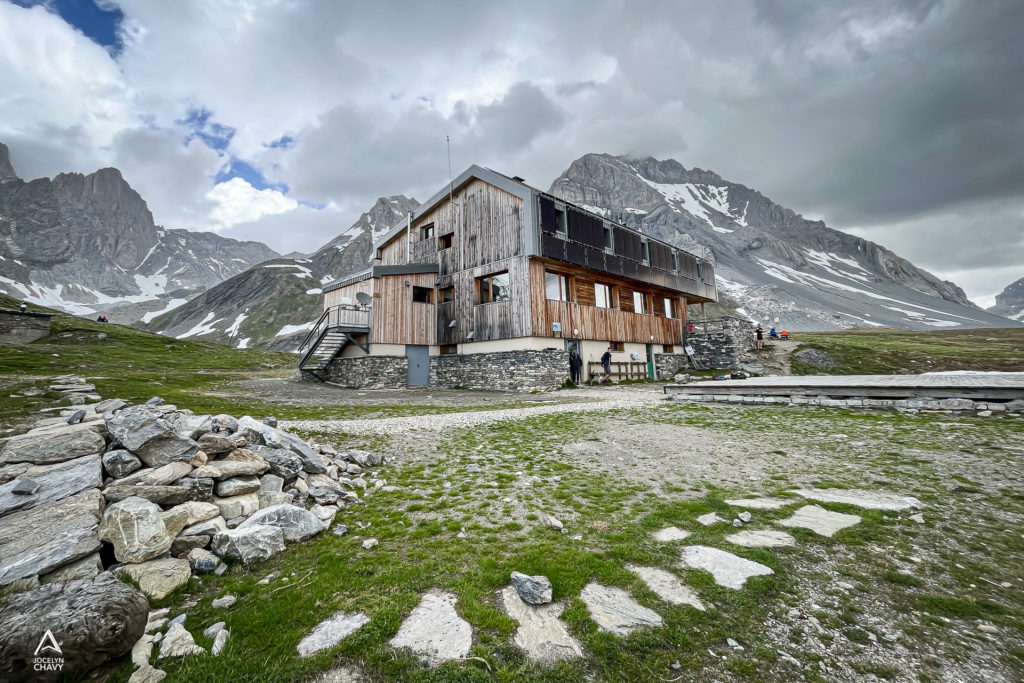The photograph captures a striking scene dominated by a sky filled with fluffy, storm-like clouds tinged with gray, suggesting imminent rain, while a sliver of blue peeks through on the left. Towering, snow-capped mountains form an impressive backdrop, emphasizing the rugged and rocky terrain of the area. Nestled in the middle of the image is a rustic yet somewhat modern wooden structure that resembles both a barn and a house, noticeable for its multiple windows and a satellite dish. This building, characterized by brown and gray wood, has steps on the side, and at the moment, two people are seen exiting - one fully outside, the other still on the walkway. The foreground features a conspicuous pile of stones and patches of green grass interspersed with dirt, further contributing to the remote and arid feel of the location. A gravel walkway extends towards the barn from the front of the photograph, guiding the eye through this serene yet isolated mountainous landscape.